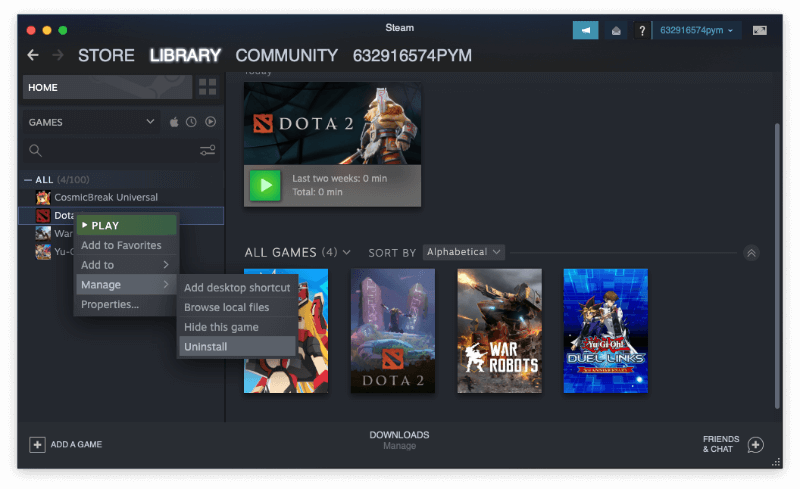The screenshot showcases a Steam games library page against a sleek black background. In the top-left corner, three small colorful circles—red, yellow, and green—are arranged horizontally. Centrally placed at the top is the word "STEAM" in small print. Directly beneath, an arrow points to the left towards the word "STORE" in larger, white text. Adjacent to it, in bold white letters, are the options "LIBRARY" and "COMMUNITY."

A vertically arranged box, starting below these tabs, contains the options "HOME" and "GAMES." Dominating the middle-right of the page is an image of the game 'DOTA 2,' featuring a warrior clad in striking armor. Just below this image, a play button is prominently displayed, accompanied by the statistics "LAST 2 WEEKS: 0 MINUTES" and "TOTAL: 0 MINUTES."

On the left side, "COSMIC BREAK UNIVERSAL" is listed beneath its play button. Below this entry, the game 'DOTA 2' reappears, also with a dedicated play button. Additional interactive options include "ADD TO FAVORITES" and the expandable "ADD TO" and "MANAGE" menus. The "MANAGE" menu, highlighted with an arrow, lists "ADD DESKTOP SHORTCUT," "BROWSE LOCAL FILES," "HIDE THIS GAME," and highlighted on the list is "UNINSTALL."

Towards the bottom of the page, four game covers are displayed, though one is partially obscured. The visible covers are 'DOTA 2,' followed by 'WAR ROBOTS' and 'YU-GI-OH DUEL LINKS.'